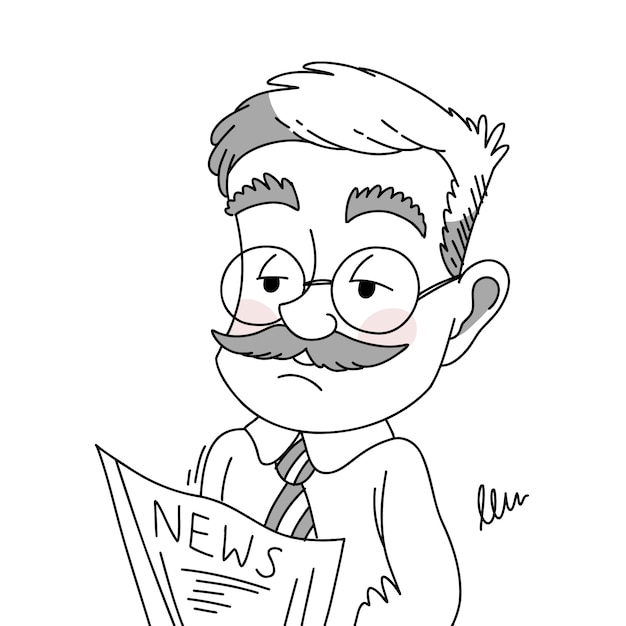This black-and-white and gray illustration features a 50-year-old man with distinctive facial characteristics, including thick, bushy eyebrows, a bushy mustache, and rosy pink cheeks—the only color in this simple line drawing. He is wearing round eyeglasses that frame his eyes as he looks towards the left, and is dressed in a white shirt paired with a gray and white striped tie. The man's hair is short, with gray on one side and white on the other, complemented by matching gray sideburns. He holds a piece of paper labeled "news" close to his face, suggestive of reading a newspaper, though it's unclear if he's standing or sitting. A cursive signature, possibly "LLU," appears at the bottom right of the illustration. The overall style is cartoony and straightforward, with minimal detail except for the signature and the man's expressive facial features.